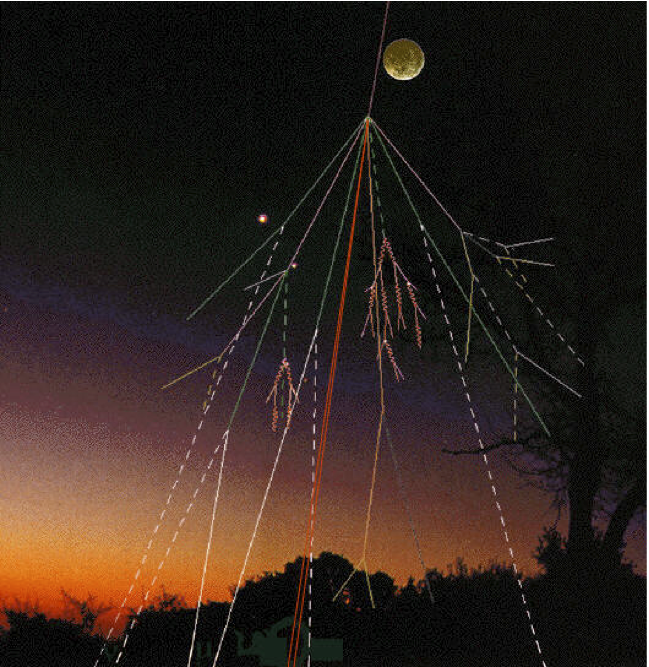This image captures a serene outdoor scene at dusk, showcasing a graduated color palette that transitions from a deep orange near the horizon to a lighter orange, then purple, navy blue, and finally black at the top, indicating either sunrise or sunset. The moon is prominently visible in the sky, casting a subtle glow over the landscape. Below, a silhouette of a tree line is rendered in black due to the low light, with a larger tree standing tall on the right side. Superimposed on this tranquil setting, several digital elements are evident: multiple laser-like lines in red, green, and white extend vertically from the bottom edge to just beneath the moon, creating a dynamic overlay. Dotted white lines further add to the composition, suggesting a possible diagram or digital enhancement that contrasts with the natural beauty of the scene.